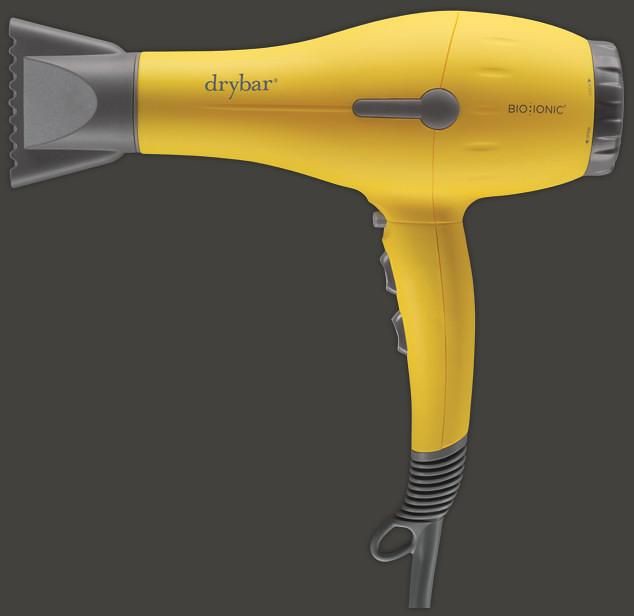The image is a highly detailed, hyper-realistic depiction, likely computer-generated, of a banana yellow Bio-Ionic Drybar hair dryer set against a charcoal gray background. The hair dryer is positioned in a side view, with its nozzle facing out to the left. The device features a prominent yellow body with black accents, including the cord, motor housing, and nozzle. The bottom center of the image reveals part of the black cord and a rubbery black end at the handle’s base. 

Three black buttons are seen on the left-hand side of the handle. The main body, marked with "Drybar" in gray lettering, extends horizontally, with a back end featuring a black exhaust area and a black dial for adjusting settings. The front nozzle has a unique design with white, wavy diffuser lines ending in a comb-like structure, which facilitates hair drying and styling. The overall design also includes a gray switch located above the neck and additional buttons on the midsection of the dryer, possibly for adjusting temperature and speed settings.